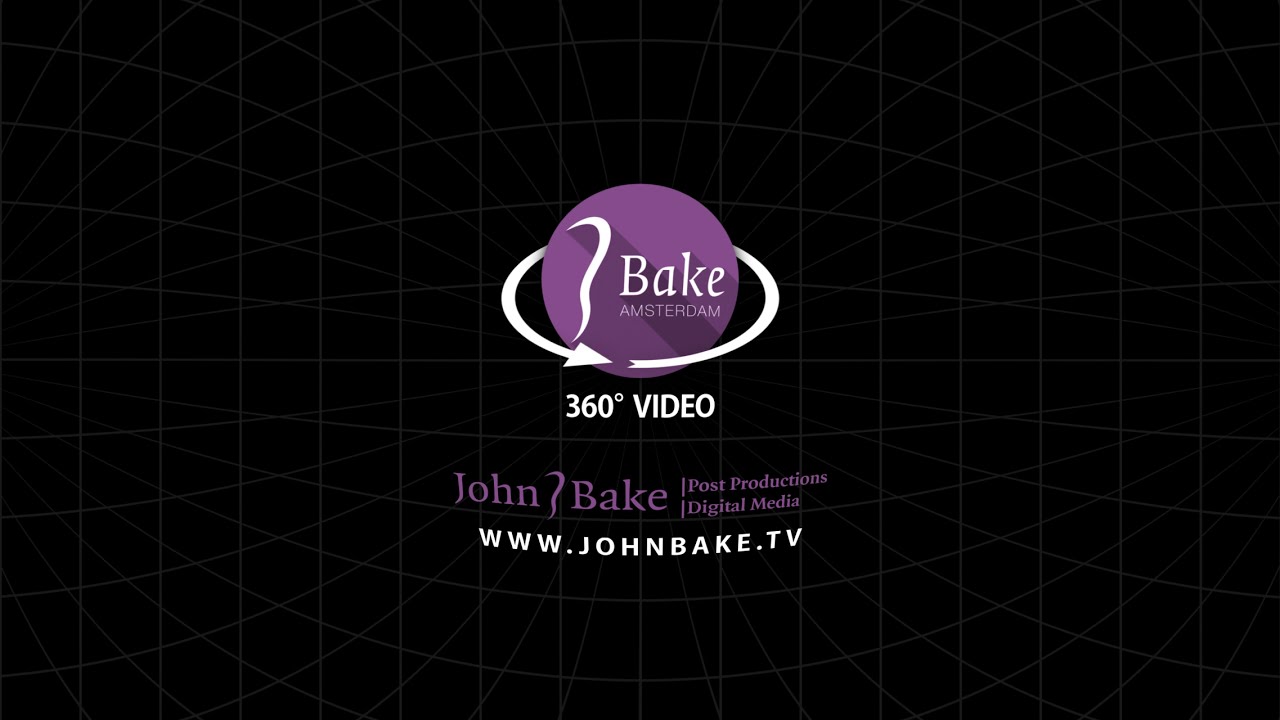The image features a digitally created rectangular poster with a predominantly black background. Subtle, faint gray grid lines curve and warp vertically and horizontally, creating a modern, abstract wireframe design. At the center of this black and white grid is a prominent blue-purple circle surrounded by a white, orbiting arrow. Inside the circle, in white text, are the words "Bake Amsterdam," and next to them is a character resembling an earlobe or a question mark. Beneath this central circle, in bold white text, it reads "360 DEGREE VIDEO." Further down, the text "John," followed by the earlobe-like symbol, "Bake," and "Post-Production Digital Media" appear in purple. At the very bottom of the image, in white text, the website "www.johnbake.tv" is displayed. The composition is highly focused, with the central elements standing out against the minimalist, black grid background.